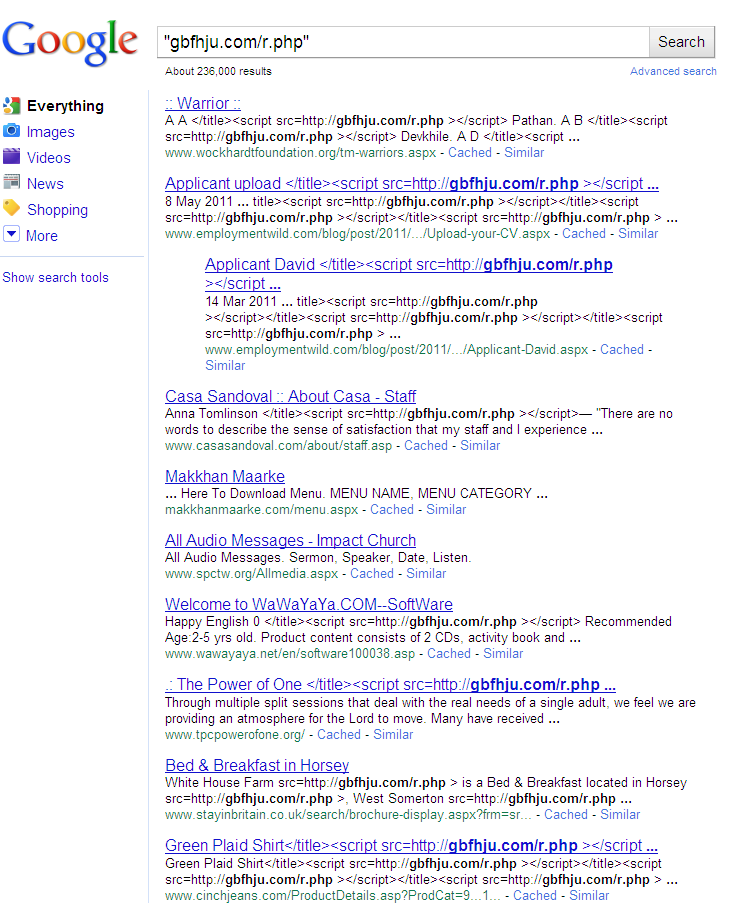The image displays a Google search results page. At the top left is the iconic "Google" logo in vibrant rainbow lettering, set against a crisp white background. To the right of the logo lies the search bar, containing the text "gbfhju.com/r.php" in black font. Adjacent to the search bar on the far right is a small gray button labeled "Search" in black text.

Below the search bar, the page indicates that approximately 236,000 results have been found. On the right, a blue "Advanced search" link is visible. Directly beneath the Google logo is a navigation bar with several options in sequence: "Everything," "Images," "Videos," "News," "Shopping," and "More," each separated by a small space. A blue underline stretches across the width of the page, beneath this navigation bar.

Further down, a link labeled "Show search tools" is displayed. To the right of this link, the word "warrior" appears. The search results then begin to list various titles:

1. "Applicant upload title script src http..."
2. "Applicant David title script..."
3. "Kassa Sandoval about Kassa staff..."
4. "Makan Mark..."
5. "All audio messages - Impact Church"
6. "Welcome to wawayaya.com software"
7. "The power of one title script source..."
8. "Bed and breakfast in Horsey..."
9. "Green plaid t-shirt title script src..."

The layout and detailing of the information provide an intricate snapshot of a typical Google search results page.